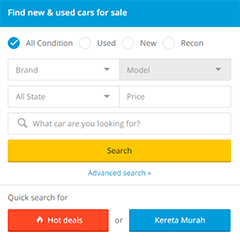In the image, we observe a blurred roster advertising new and used cars for sale, prominently displayed on a blue banner with crisp white lettering. Directly beneath this banner is a blue checkmark icon, highlighting clickable choices labeled "All Condition," "Used," "New," and "Recon." Below these options, a series of dropdown menus are visible, with labels for "Brand," "State," "Price," and "Model." The "Model" dropdown appears shaded in gray, indicating it is either selected or available for user interaction.

Further down, there is a prompt asking, "What car are you looking for?" accompanied by an hourglass icon as a choice, suggesting a search feature. Beneath this prompt is a conspicuous yellow search bar with the word "Search" prominently displayed within it. Adjacent to the search bar, a white box with blue lettering reads "Advanced Search," offering more specific search parameters for the user. Just below, another section titled "Quick Search" features two distinct buttons: one, labeled "Hot Deals," is a bright red button emblazoned with what appears to be half of a white flame icon, signifying exclusive offers. To the right of this button, there is another box labeled "Coretta Murrah" in a bright blue with blurred white lettering, indicating another searchable category or option.

The overall layout appears user-friendly, designed to facilitate an efficient and streamlined car search experience.